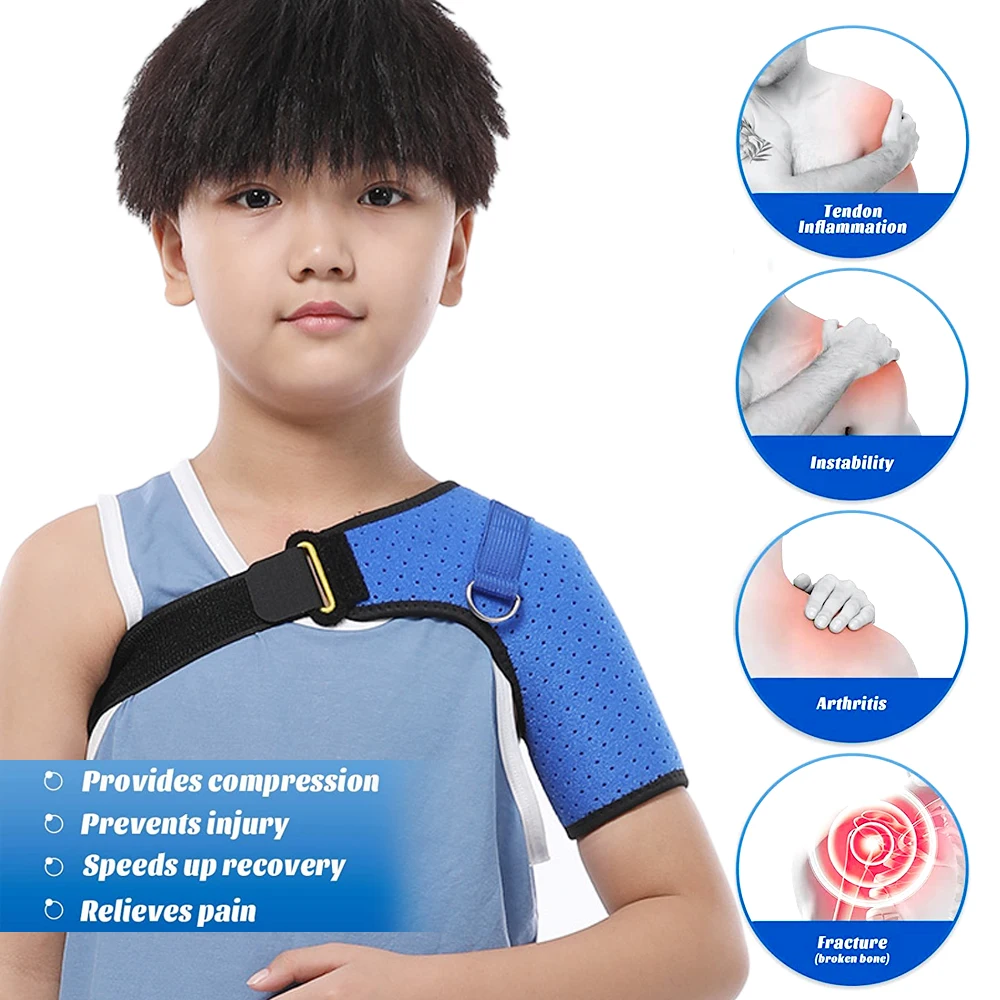This image appears to be an advertisement featuring a young boy, probably under 10 years old, with an Asian appearance, light tannish skin, dark eyes, and thick dark brown hair. He is wearing a light blue tank top and a blue sling or compression brace on his right shoulder, which extends around his body to under his left arm, secured with a Velcro strap. The background is white. On the left side of the image, there is text stating, "Provides compression, prevents injury, speeds up recovery, and relieves pain." To the right of the boy are four circles illustrating different shoulder conditions with varying degrees of redness indicating inflammation and pain. The conditions shown are Tendon Inflammation, Instability, Arthritis, and Fracture, each depicted with a relevant visual and label. The image conveys how the sling helps mitigate these conditions.